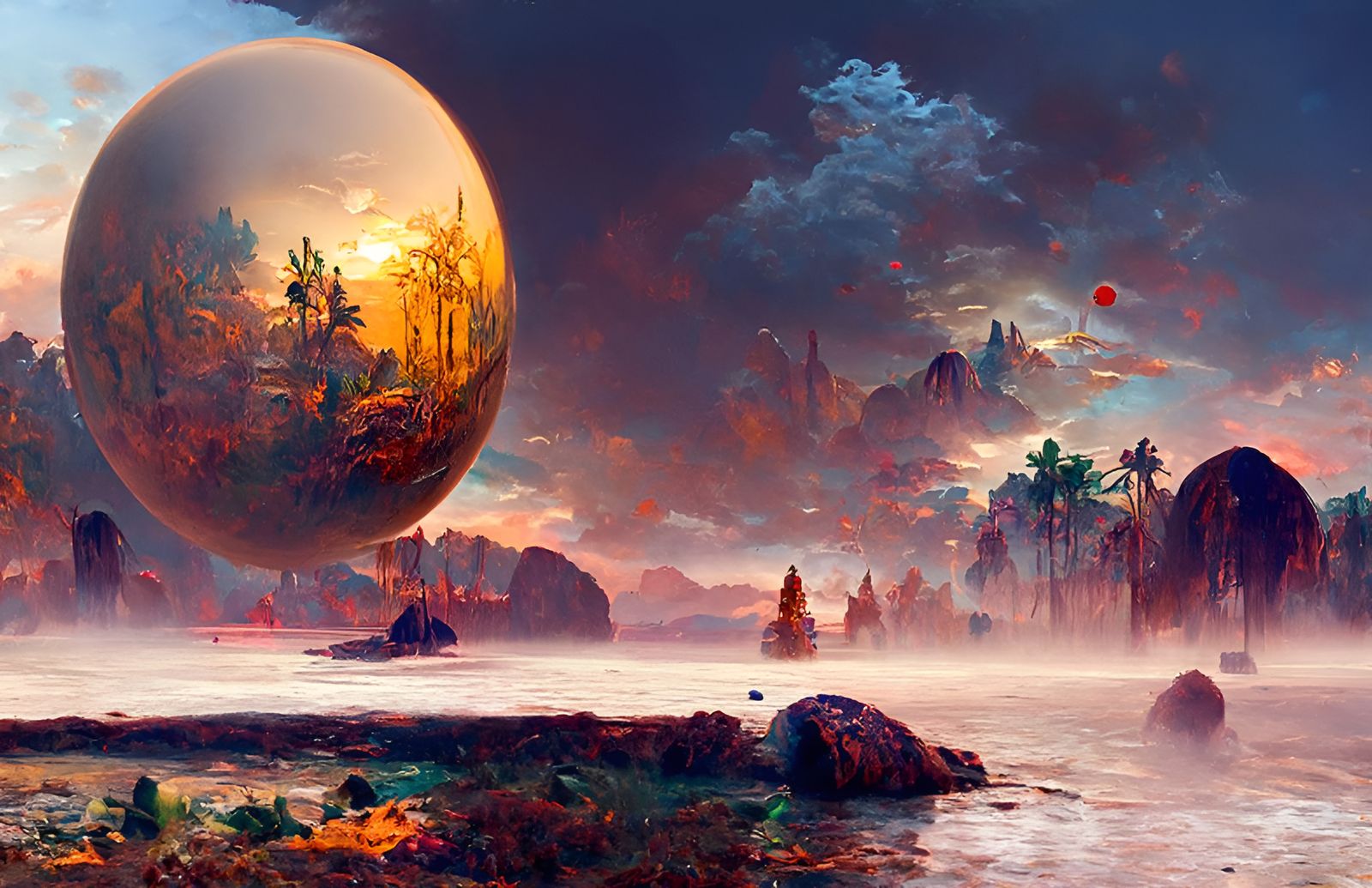This digital artwork presents a stylized vision of a futuristic, faraway planet drenched in an array of vibrant colors, from deep and lighter blues to amber, gold, wine, and touches of green. Dominating the composition, a large amber sphere floats near the left side, mirroring the multicolored vegetation and scenery around it. Below the sphere lies a small, green lake shrouded in a slight mist, with a rocky, craggy beach featuring scattered greenery and flowers stretching from the lower left corner to the middle of the image.

In the distance, towering rock formations ascend into the sky, alongside palm tree-like flora. The skyline transitions from light blue on the left to a stormy black atmosphere with light blue clouds, adding a sense of mystery. The reflective lake is bordered by a ridgeline of rocks and trees, while above, a star, sun, or planet in striking red hue hovers amidst the sky. This intricate and immersive scene evokes an otherworldly landscape, blending elements of rocky textures, water bodies, and surreal vegetation under a stunningly dynamic sky.